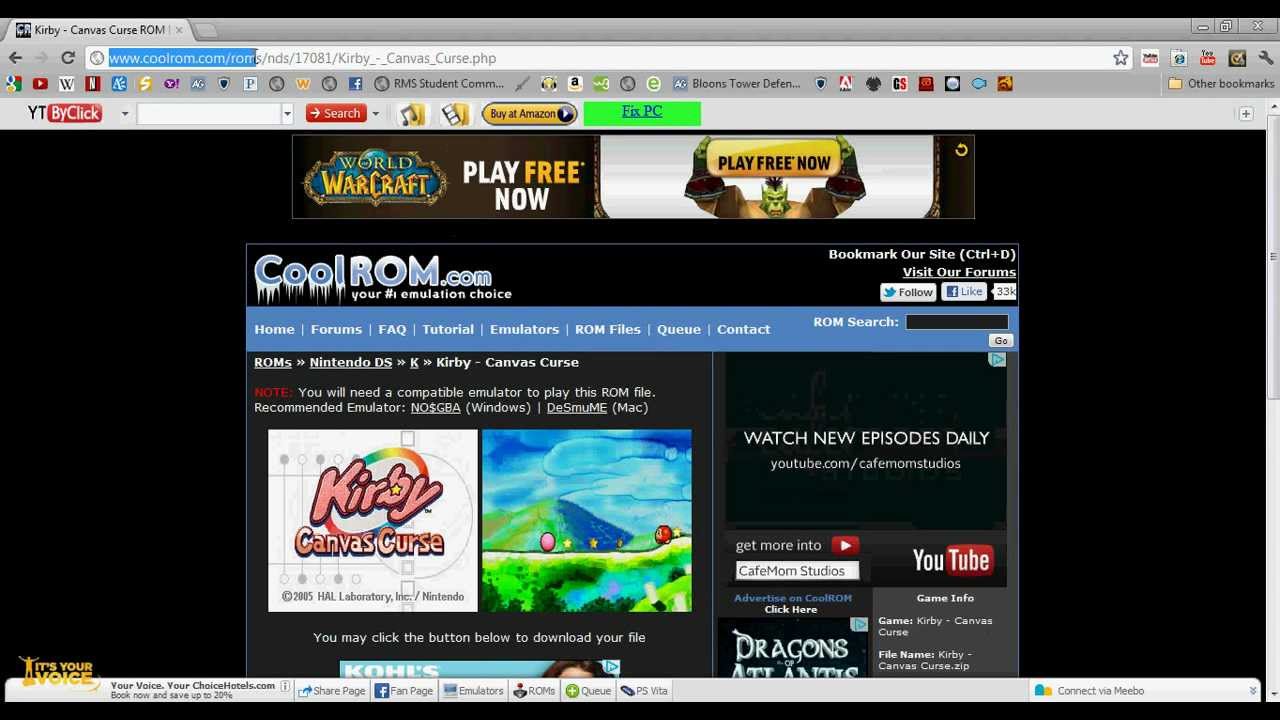The screenshot captures a browser window with a single tab open, displaying the website "coolrom.com." The browser appears to be an older version, possibly from Chrome or Internet Explorer, characterized by an array of icons and shortcuts at the top. These include bookmarks and quick-access buttons, such as "YT by Click," a dropdown menu, a search button, and options like "Buy on Amazon" and "Fix PC." 

At the top of the webpage, there's an advertisement for "World of Warcraft" featuring a "Play Free Now" button. Below this, the content of the page highlights "coolrom.com" as the user's number one choice for emulation, encouraging visitors to bookmark the site and participate in its forums. The screen also contains navigational menus and additional information relevant to the site's offerings.